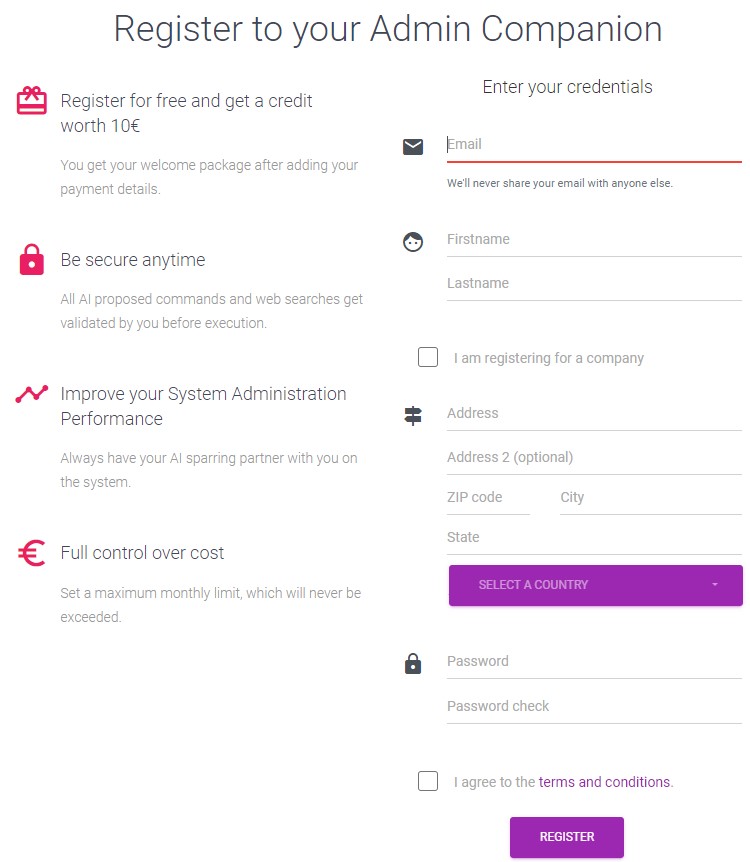The screenshot displays a registration page for an administrative companion software. At the top center, it prominently reads "Register to Your Admin Companion." The page is divided into two columns.

**Left Column:**
- **Register for Free:** Gain a £10 credit upon registering.
- **Welcome Package:** Available after adding payment details.
- **Be Secure Any Time:** All AI proposed commands and web searches require user validation before execution.
- **Improve System Administration Performance:** Keep an AI sparring partner always ready on the system.
- **Full Control Over Cost:** Set a maximum monthly limit that will never be exceeded.

**Right Column:**
- **Enter Your Credentials:**
  - **Email:** The user’s email field is highlighted, with the cursor positioned there. A note reassures users that their email will not be shared with third parties.
  - **First Name**
  - **Last Name**
  - **Checkbox:** Option to register for a company.
  - **Address Lines (two fields)**
  - **Zip Code**
  - **City**
  - **State**
  - **Country:** A drop-down box currently displayed in purple.
  - **Password:** Field to enter a password, followed by a "Password Check" field to re-enter the password for confirmation.
  - **Terms and Conditions:** A checkbox to agree to the terms and conditions, with the terms and conditions hyperlink highlighted in purple.
  - **Register Button:** A purple button with white text that says "Register."

This comprehensive layout ensures users know exactly what to expect and how to proceed with their registration.